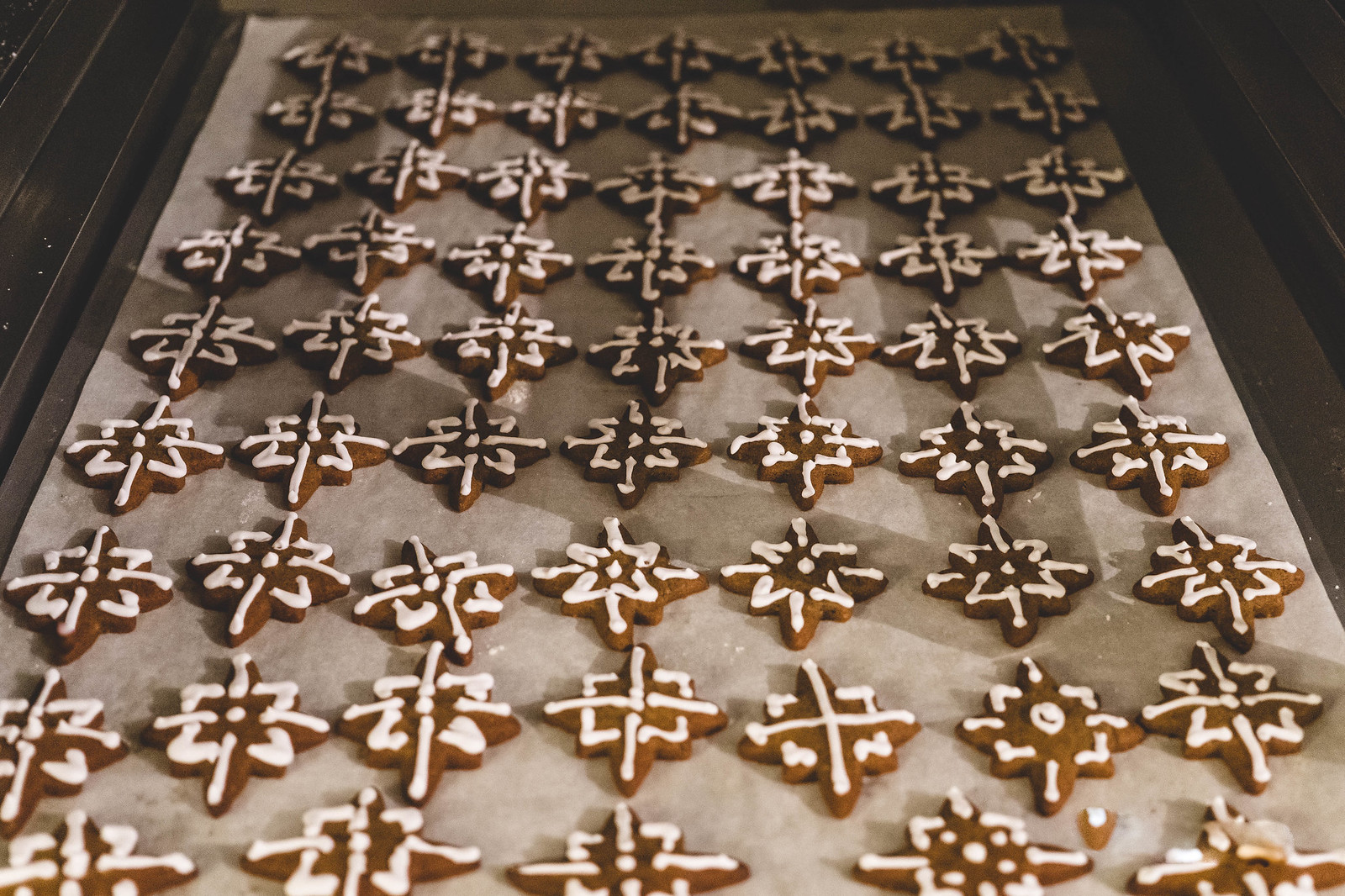This is an image of a large batch of small, homemade cookies arranged on a black parchment-lined baking sheet. The cookies, possibly gingerbread, are uniformly brown and shaped like stars, some resembling North Stars. Each cookie is intricately decorated with white frosting, featuring patterns such as stars, crosses, dots, and diamond shapes, resembling snowflakes or symmetrical designs. There are approximately seven rows of nine cookies each, creating a visually appealing display that looks freshly baked and meticulously crafted.